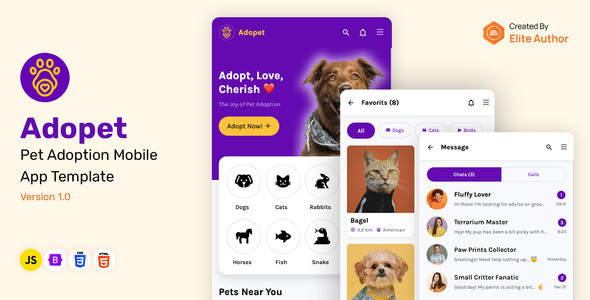This is a caption that someone provided for an image using their voice. I've cleaned it up and formulated it into a detailed descriptive caption:

---

This image showcases a template from the Adopt-o-Pet mobile app, version 1.0, designed for pet adoption. In the upper section, there's an icon labeled "JS" along with several other icons. At the center of the page, a card featuring a dog with a bandana around its neck is prominently displayed on a purple background. The card carries the inspirational message "Adopt, Love, Cherish," accompanied by a red heart, and a call-to-action button stating "Adopt Now!" with an exclamation point.

The app categorizes pets into various sections where users can click to explore dogs, cats, rabbits, horses, fish, and snakes. Towards the bottom, the section labeled "Pets Near You" is visible, though partially cut off. Within this section, there is a card showing a cat named Bagel, while a dog is pictured beneath it, but its name is not fully visible.

Additionally, the app features an interactive messaging area with a purple slider. Currently, one side is highlighted but not the other. Categories such as "Fluffy Lover," "Terrarium Master," "Paw Prints Collector," and "Small Critter Fanatic" are also displayed, indicating different user preferences or badges.

---

This detailed caption provides a comprehensive overview of the app template layout and content.